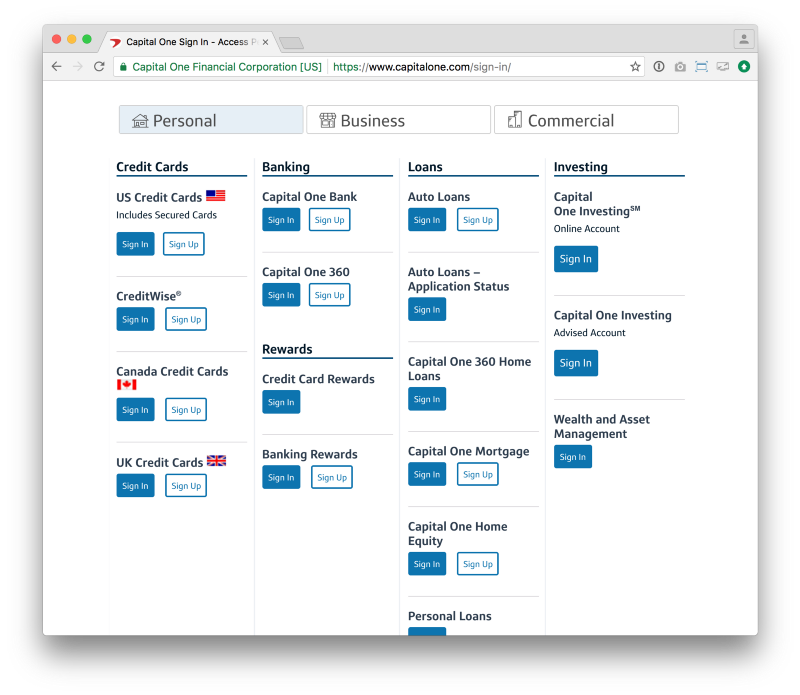The image depicts a screenshot of a Capital One website, showcasing various menus and options for user sign-ins and account access. The top left corner features a series of three dots—red, yellow, and green—typically representing window control buttons on a computer screen. Below this, the browser’s address bar displays a URL in green and gray fonts: “Capital One Financial Corporation [U.S.]” followed by “https://www.capitalone.com/sign-in/”.

The main navigation menu at the top is divided into three sections: “Personal”, “Business”, and “Commercial”, each with corresponding icons. The “Personal” section is highlighted in light blue, indicating it is currently selected.

Below this, there are several sub-menus:
1. **Credit Cards**: Includes options such as "U.S. Credit Cards" marked with an American flag, "Include Secured Cards", and two horizontal buttons—one turquoise with "Sign In" in white font, and the other white with a turquoise border and "Sign Up" in turquoise font.
2. **CreditWise**: Offers sign-in and sign-up options.
3. **Canada Credit Cards**: Displayed with a Canadian flag, offering sign-in and sign-up options.
4. **UK Credit Cards**: Displayed with a UK flag, offering sign-in and sign-up options.

Next is the **Banking** category, featuring:
- Capital One Bank
- Capital One 360, both with sign-in and sign-up buttons.

The **Rewards** section includes:
- Credit Card Rewards: Sign in
- Banking Rewards: Sign in and sign up

The **Loans** category lists multiple options:
- Auto Loans: Sign in and sign up
- Auto Loans Application Status: Sign in
- Capital One 360 Home Loans: Sign in
- Capital One Mortgage, Capital One Home Equity: Both with sign-in and sign-up
- Personal Loans: Sign in

Finally, the **Investing** category features:
- Capital One Investing
- Online Account (Sign in)
- Capital One Investing (Advised Account) (Sign in)
- Wealth and Asset Management (Sign in)